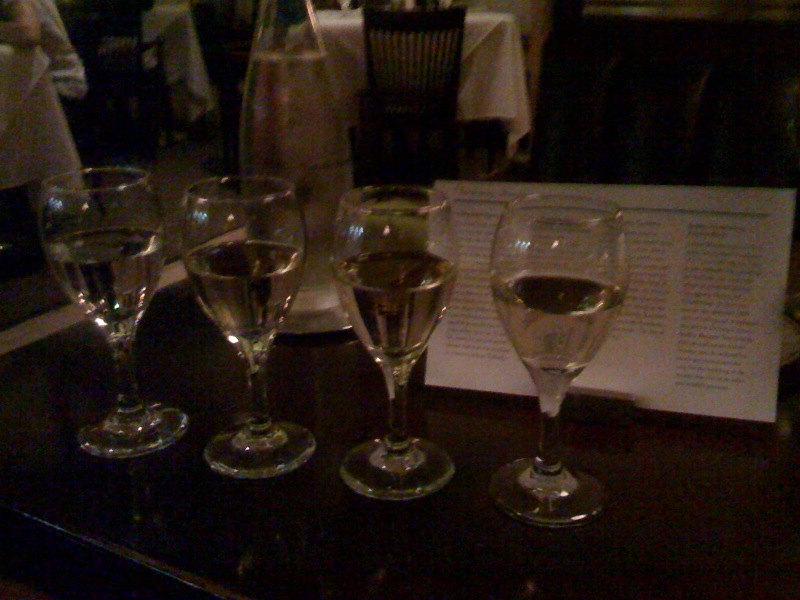The image is a realistic photograph with a horizontal rectangle shape. Despite the slightly dark lighting, we can discern a restaurant or banquet hall interior. The background features several square tables adorned with white tablecloths that have tiny yellow flowers, paired with dark brown or black chairs. Amidst these, partially obscured, is a figure or a chef in a white jacket, or possibly just another table with a person’s elbow visible.

In the foreground, a dark brown, possibly wooden, table shines with a polished surface. On this table, there are four crystal wine glasses, each filled about halfway with a clear, transparent liquid, potentially wine or champagne, and adorned with gold trim on their rims. Behind these glasses to the left stands a tall clear glass, possibly containing water, and a clear bottle with liquid. To the back right, a horizontal white card with black text is visible, though its text is too small and dark to be legible.